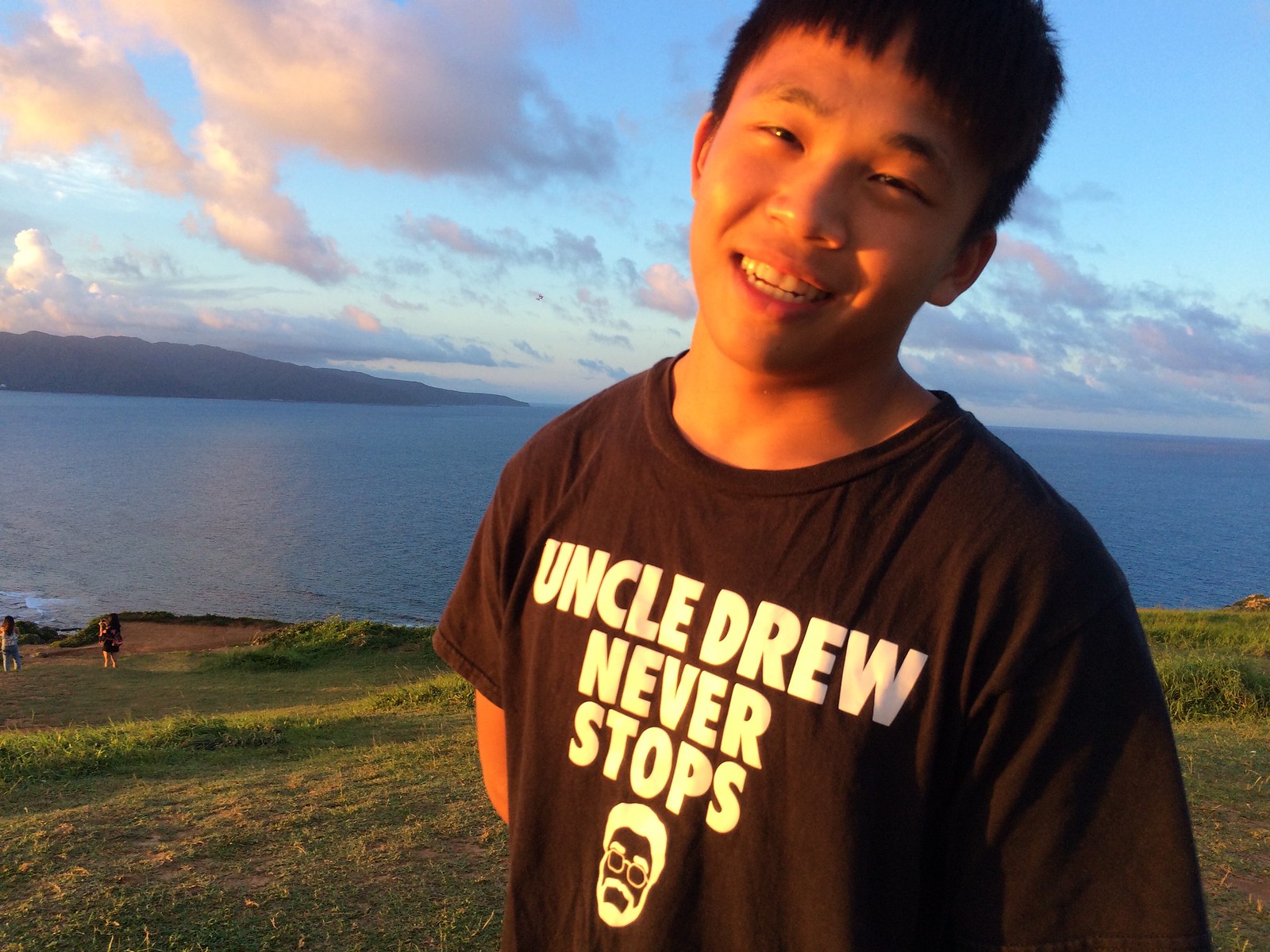The photograph captures a young man of Asian descent standing confidently on a grassy hillside under a clear, bright blue sky, with the soft hues of an orangey-pink sunset illuminating his face. The sun is setting from the left side of the image, casting a warm glow across the scene. Behind him stretches a vast body of water, possibly a large lake or the ocean, extending to the horizon where small mountains or large hills rise up, creating a natural backdrop. The shoreline in the distance features a few people facing the water, adding depth to the serene landscape. The young man stands near the forefront, almost occupying half the frame, smiling directly at the camera. He is wearing a black t-shirt with bold white text reading "Uncle Drew Never Stops," accompanied by a caricature of Uncle Drew, a character known from basketball commercials. The image beautifully blends the striking natural panorama with a personal, posed portrait, emphasizing both the scenic sunset and the young man’s cheerful demeanor.